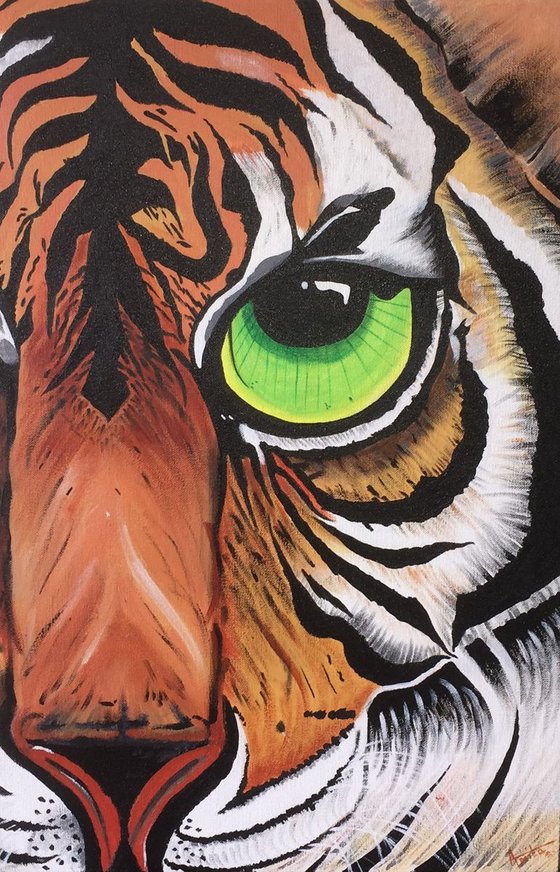This close-up, vertically oriented graphic image portrays the striking face of a tiger. Dominating the left side of the image is the tiger's prominent nose, detailed with distinguishing arches and flanked by patches of white fur. Surrounding the nose, brown fur seamlessly transitions into the visage of the tiger. The most captivating feature is a single, large green eye located prominently within the frame, exhibiting intricate lines on the eyeball that enhance its realism. The other eye is partially obscured, extending beyond the left edge of the image.

The upper portion of the tiger’s face is adorned with a pattern of black and brown stripes, interspersed with white spots, all resembling the authentic texture of a tiger’s fur. These stripes form rounded shapes that extend beneath the visible eye and create a cascading effect. Adding to the lifelike quality, fine white whiskers sprout from the side of the mouth, accentuating the tiger’s muzzle.

Despite its realism, the image carries an abstract touch with vibrant and diverse colors, making it both a visually arresting and artistically nuanced depiction of the majestic tiger.